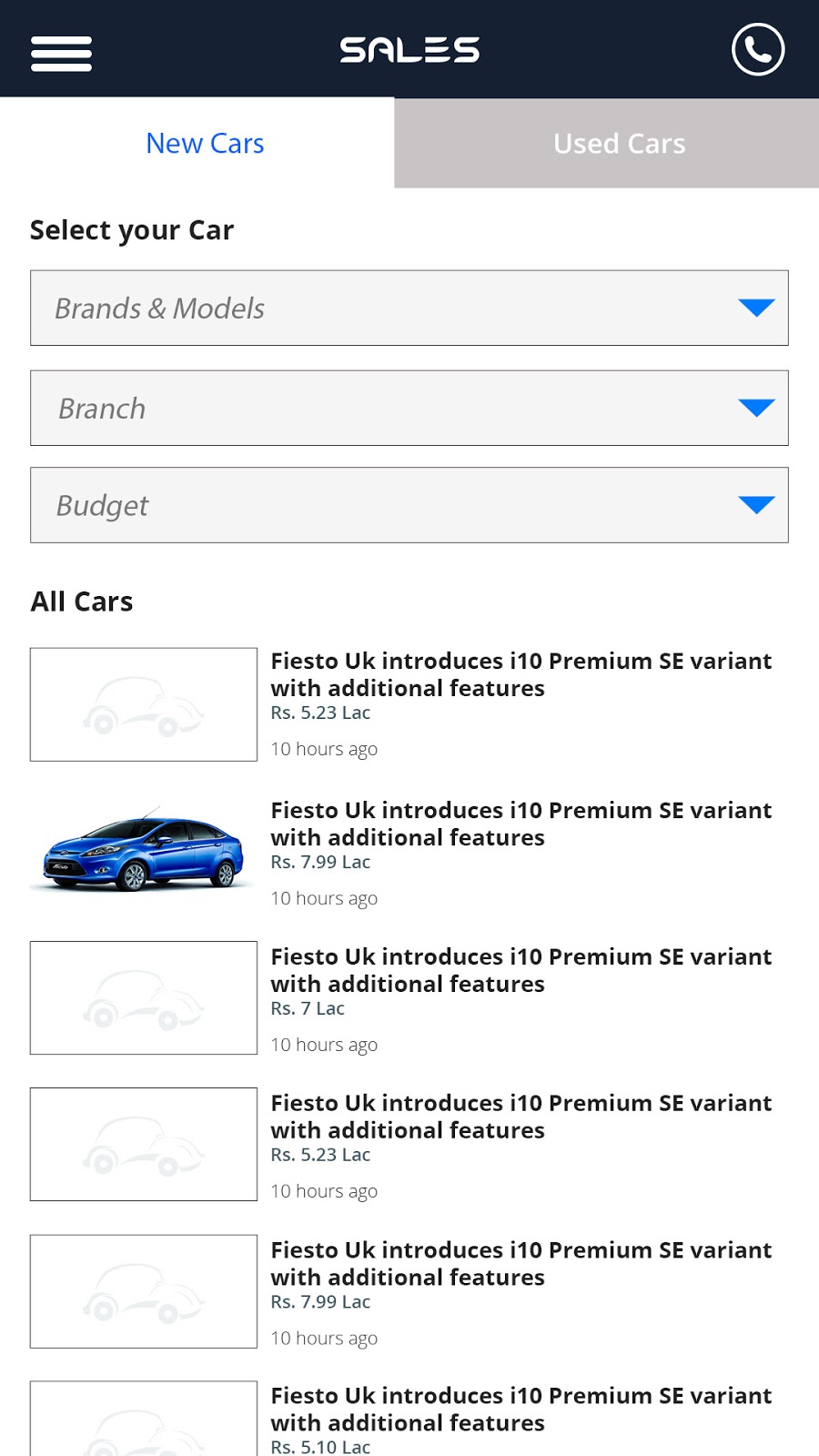The image depicts a car sales app interface, prominently featuring the word "Sales" at the top. Adjacent to the title, there is a circular icon with a phone symbol, and to the left, three horizontal lines of equal length, possibly representing a menu. 

Below these icons, the interface categorizes vehicles with buttons labeled "New cars" in blue font and "Used cars" in white font on a gray background. The app prompts users to "Select your car" with options to filter by "Brands and Models," "Branch," and "Budget," each accompanied by a blue downward arrow for dropdown selection.

Displayed on the screen is a section titled "All Cars," featuring a black and white box with the image of a car. Beneath this, a headline announces "Fiesto UK introduces i10 Premium SE variant with additional features." Following this, there's an image of a blue car oriented to the left with the same announcement text repeated.

This layout and announcement are duplicated for four other cars, each illustrated in black and white with identical repeating text.